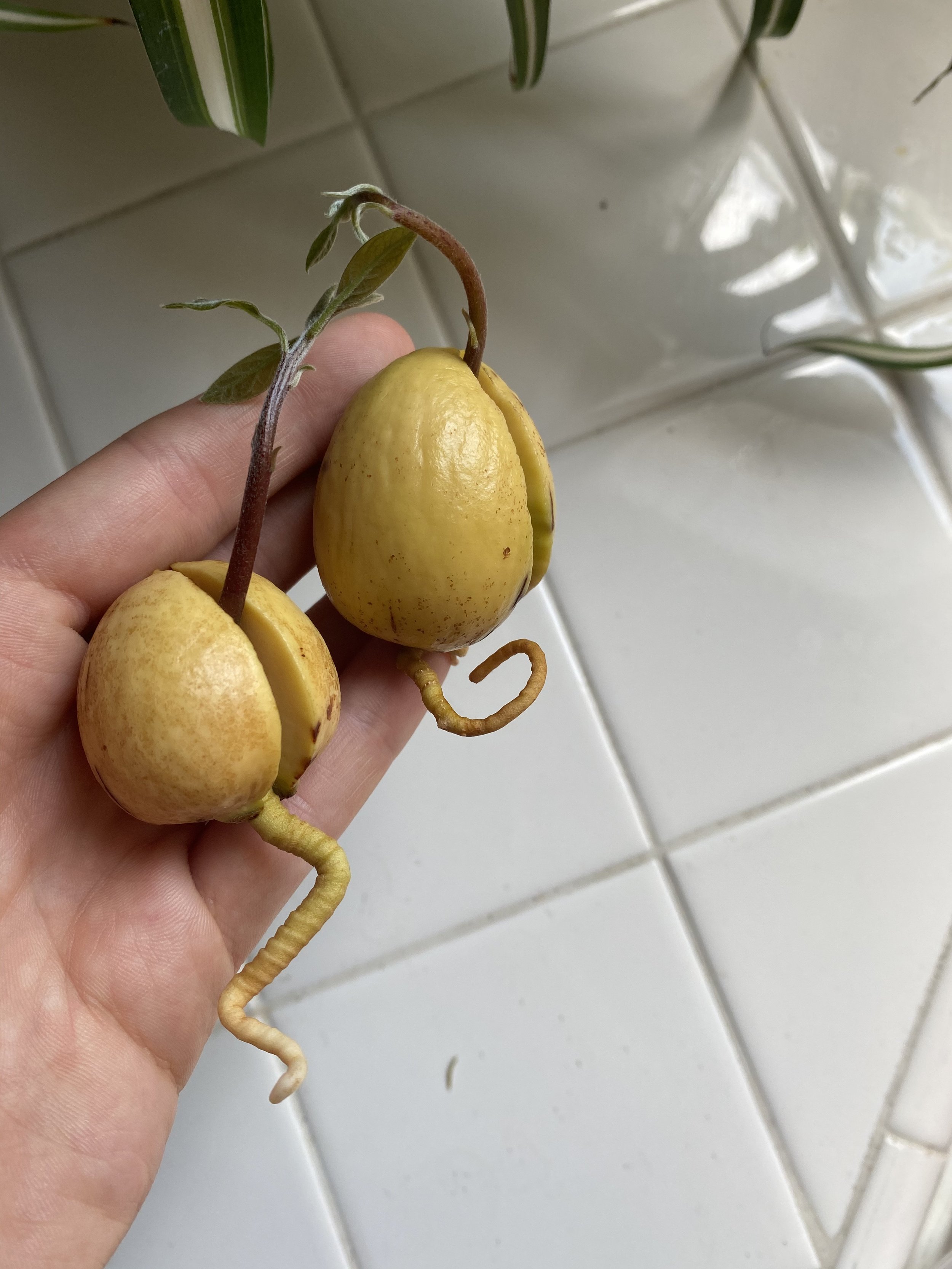This indoor photograph captures the partial view of a person's left hand, positioned on the left side of the image, holding two avocado pits. The pits are yellowish-green, almost olive in color, and have split open in the middle. From the bottom of each pit grows a long, curly yellow root, while from the top emerge reddish-brown stems adorned with green leaves. The pit on the left features a longer stem, root, and more numerous, larger leaves compared to the pit on the right. The background reveals a shiny, reflective tile countertop with mostly white square tiles and some triangular ones. Additional green leaves droop from a nearby house plant at the top of the image, complementing the scene.